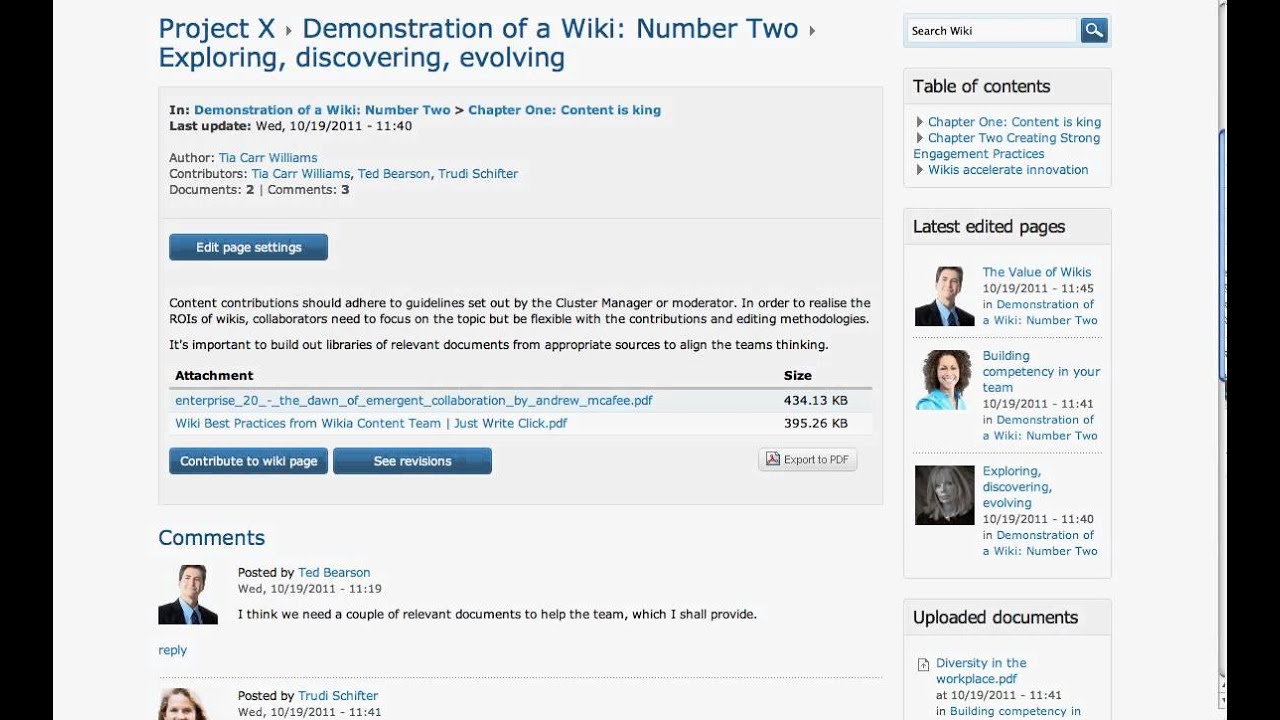This is a screenshot of a website featuring a wiki forum. The image has two black bars on either side, with the webpage itself being off-white. At the top, the header reads, "Project X → Demonstration of a Wiki: Number Two → Exploring, Discovering, Evolving." The layout suggests that it is structured like a forum.

On the right side of the webpage, there is a search bar labeled "Search Wiki." Below this, a "Table of Contents" is displayed, listing various chapters. This section also includes "Latest Edited Pages," showing icons of users along with the articles they have edited and uploaded documents.

In the main body of the page, under "Demonstration of a Wiki: Number Two, Chapter One: Content is King," details about the chapter are provided, including the last update date, author's name, contributor names, document numbers, and comment numbers. There is a notable blue button labeled "Edit Page Settings." Below this section, the text of the chapter is present, along with two attachments that can be clicked on, with their sizes indicated to the right.

Additional buttons such as "Contribute to Wiki Page," "See Revisions," and "Export to PDF" are present. At the bottom of the page, the comments section shows at least two comments. Each comment displays the user’s picture, the name of the person who posted it, the comment text, and options to reply.